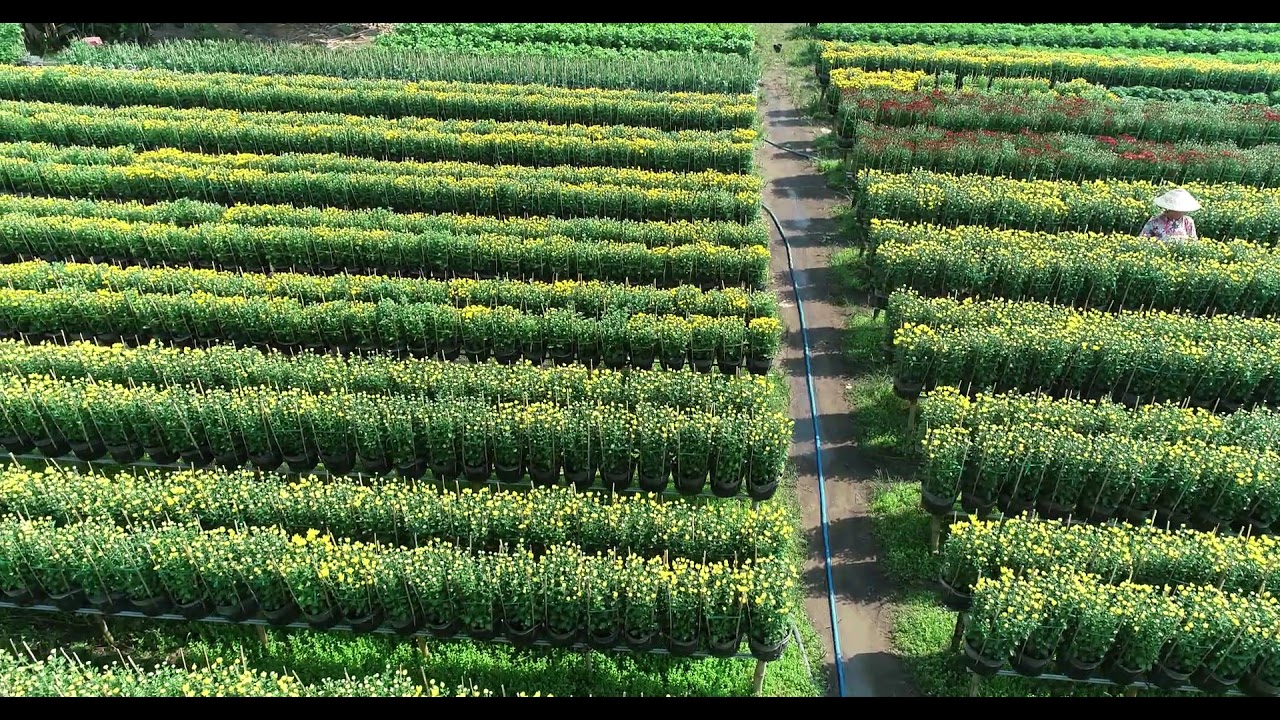The photograph depicts a well-organized, outdoor farming scene, captured during the day from a slightly elevated vantage point. Central to the image is a brown, dirt walkway that runs slightly left of the center, intersected by blue hoses that trace parts of its path. Flanking this walkway are long, raised platforms housing rows of plants in black pots. These plants predominantly display green leaves and yellow flowers, although near the top-right corner, the flowers shift to a red hue. Towards the top of the image, patches of the plants are devoid of flowers, showcasing only their verdant leaves. 

Standing partially obscured on the right-hand side of the image, between two rows of the flowering plants, is an individual dressed in a white and pink patterned shirt and sporting a traditional rice paddy hat. The hat, often associated with Vietnamese farmers, adds a cultural touch to the scene. The light suggests shadows stretching towards the left, indicating the sun is shining from the right side. The overall ambiance suggests a serene, methodical farming environment with a mix of flowering and leafy green plants.